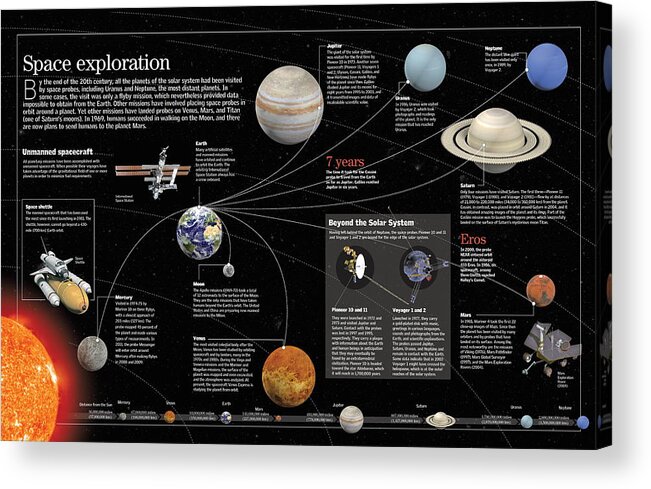The poster is a comprehensive illustration on space exploration, set against a black background filled with stars. At the top left, it features the title "Space Exploration" in bold white text. Beneath this, a detailed narrative explains that by the end of the 20th century, all the planets in the solar system were visited by space probes. This includes Uranus and Neptune, the most distant planets, with some missions being mere flybys that still provided valuable data. Other missions involved placing probes in orbit or landing them on planets like Venus, Mars, and Titan, one of Saturn's moons. It highlights the milestone of humans walking on the moon in 1969 and mentions future plans for manned missions to Mars.

The poster is adorned with images and charts. From left to right, it illustrates the Sun, Mercury, Venus, Earth, the Moon, Mars, Jupiter, Saturn, Uranus, and Neptune. There is also a section titled "Beyond the Solar System" with pictures of Pioneer 10, Pioneer 11, Voyager 1, and Voyager 2. A chart displays the relative sizes of the various planets, enhancing the visual comprehension.

There are detailed segments on unmanned spacecraft and the space shuttle, each accompanied by explanatory text and pictures. A special section talks about Eros, situated beyond Neptune. Photographs of different space probes and landers are placed strategically, with a probe on the upper left and a lander on the bottom right.

In essence, the poster serves as a rich visual guide to humanity's achievements and ongoing endeavors in space exploration.